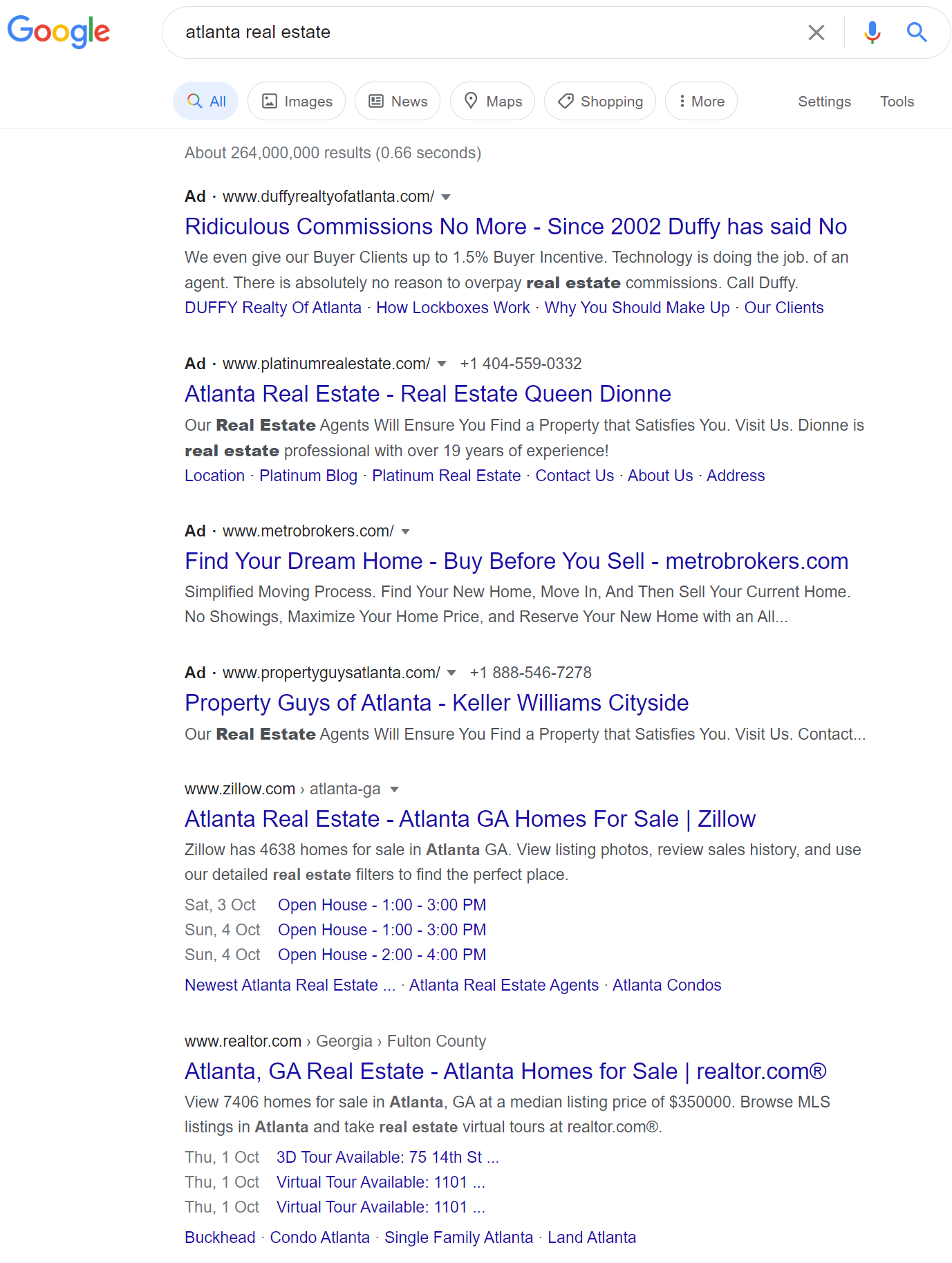The image displays a Google search results page where someone has searched for "Atlanta real estate." The "All" tab is highlighted in blue, indicating it is the active tab. The search has yielded an impressive 264 million results in approximately 0.66 seconds.

At the top of the results, a series of ads is prominently displayed. The first ad, marked by the label "Ad," directs users to "WRealtyofAtlanta.com" and touts "ridiculous commissions no more." The ad description, in standard black text, boasts of offering buyers up to a one-and-a-half percent incentive, suggesting that technology is taking over tasks traditionally performed by agents. Beneath this, another hyperlink in blue text reads, "W Realty of Atlanta: How Lockboxes Work."

Following this, the next ad links to "PlatinumRealEstate.com," which includes a phone number on the right side and the tagline "Atlanta Real Estate's Queen Deani." Two more ads appear subsequently.

Further down, organic search results begin to show up. Notably, a link to "Zillow.com" lists multiple upcoming open houses in Atlanta, providing specific dates and times: October 3rd from 1 PM to 3 PM, and the following Sunday from 1 PM to 3 PM and 2 PM to 4 PM. Finally, a link to "Realtor.com" offers 3D virtual tours for properties available starting Thursday, October 1st.